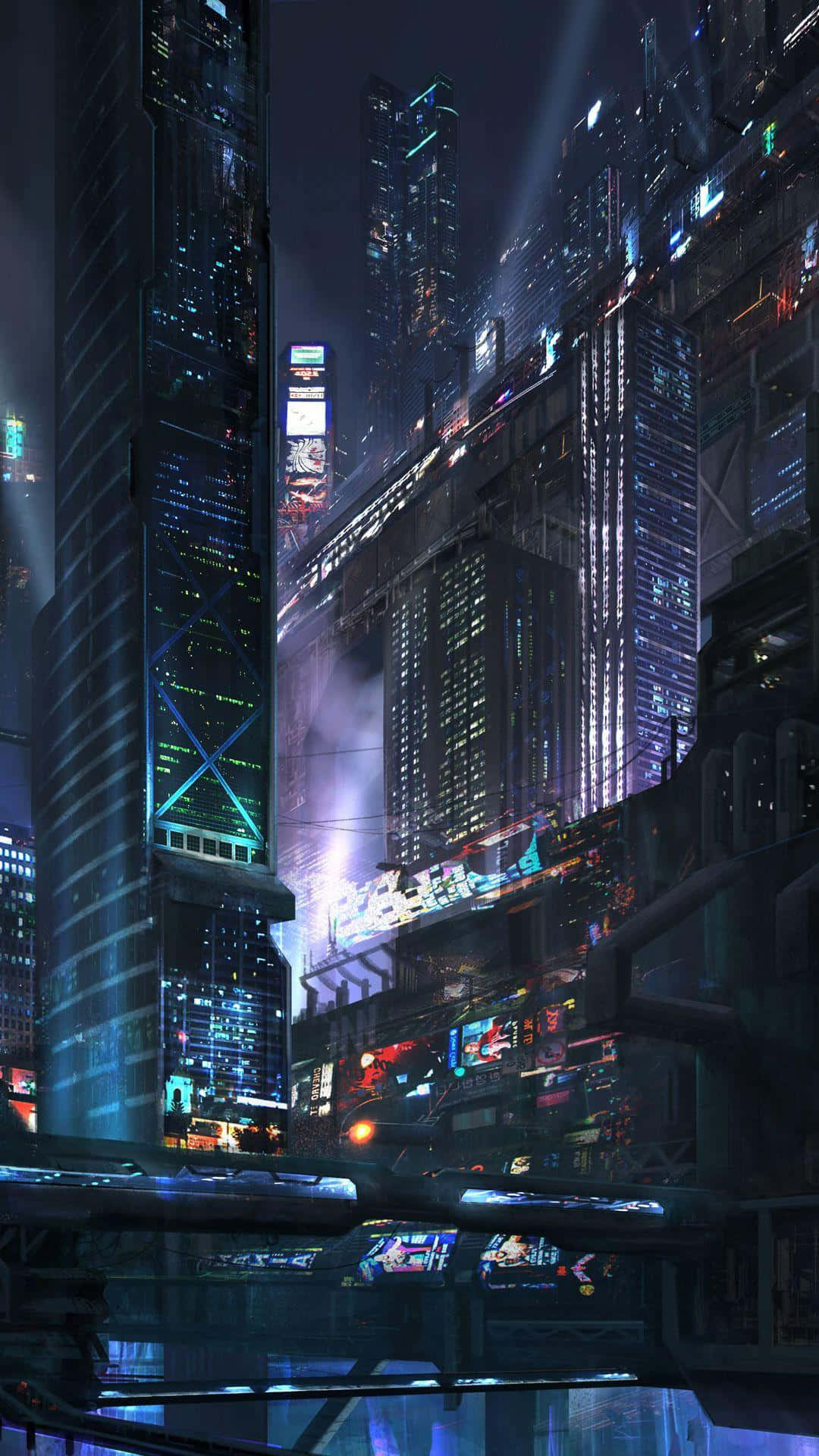The digital artwork vividly depicts a cyberpunk-style cityscape at nighttime, bathed in a purple haze. Dominating the scene are towering skyscrapers, their heights stretching out of the frame, especially one on the left. The buildings are adorned with an array of neon signs displaying vibrant reds, blues, and subtle black hues, creating a dazzling array of light. These signs are interspersed between the structures, some appearing in the foreground on an elevated bridge-like structure that cuts across the image from left to right. This rail or elevated passage connects several buildings, suggesting it might be a pathway for vehicles, possibly an elevated train. The city's myriad of windows gleam with various lights—bluish, greenish, and soft oranges—enhancing the futuristic aura. At the center of the image, a spotlight shoots a beam towards the top-right, illuminating the scene with cascading light. The overall composition suggests we are viewing the city from a lower vantage point, yet the view ascends, catching glimpses of interconnected buildings and signage fading into the misty, vertical expanse of the futuristic nocturnal skyline.